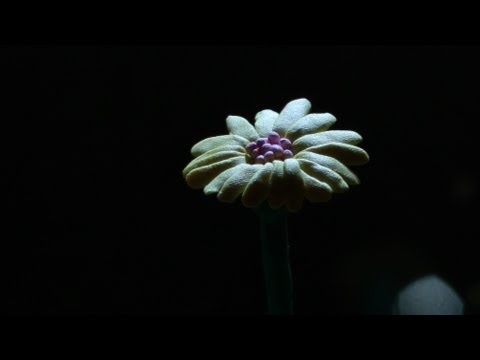The image depicts an artistic, clay-like flower bud set against a stark black backdrop, with no text or lighting. The flower's petals, appearing in shades of pinkish-white and yellow, frame the center, which features small, purplish bulbs resembling seeds or pollen. The flower is positioned slightly to the right of the image's center, with a faint outline of its green stem visible below. The bottom right corner contains a shadowy, grayish shape, although its details are blurred and partially cropped. Dark bars frame the top and bottom of the image, enhancing the overall sense of isolation and focus on the solitary, handcrafted floral subject.